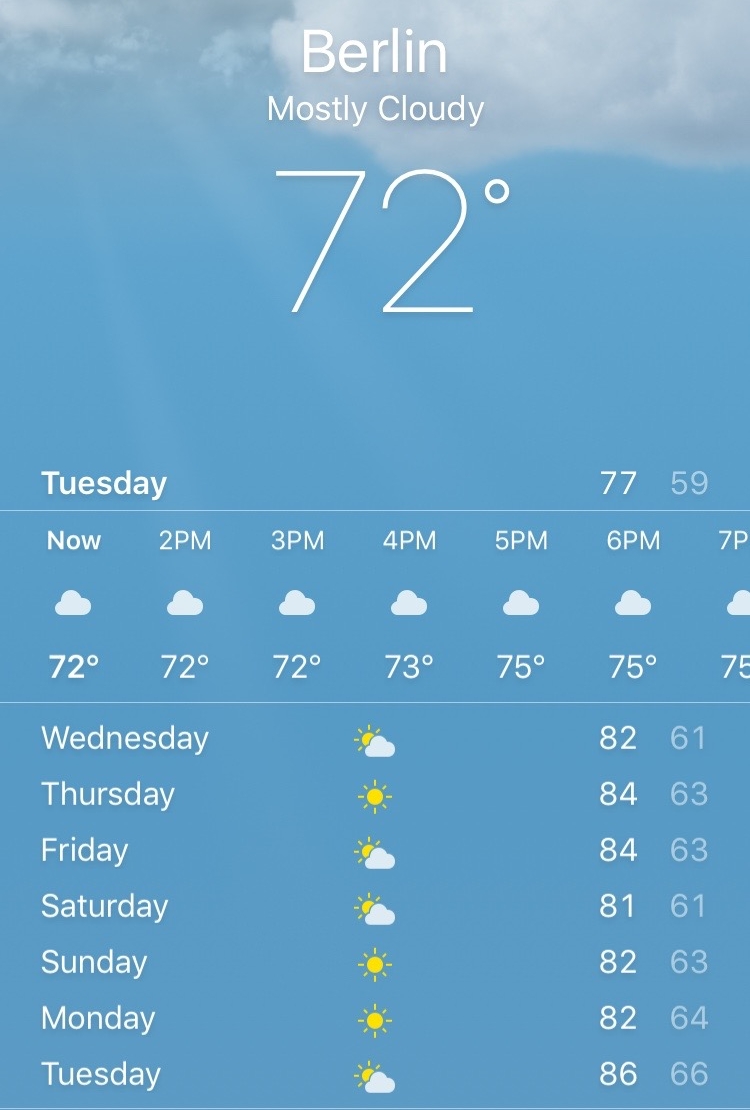A screenshot of a weather app on a mobile device, indicating the current location as Berlin with "Berlin" displayed at the top in white text. Below it, the header shows the current weather condition as "Mostly Cloudy." The primary temperature reading, in thin font, prominently displays "72°." In the background of the screenshot, a blue sky is visible with light cloud coverage at the top and sunlight peeking in from the top left corner.

The detailed weather information for the current day shows:
- "Tuesday: 77° High / 59° Low."

A timeline illustrates hourly forecasts with temperatures as follows:
- Now: 72° 
- 2 PM: 72°
- 3 PM: 72°
- 4 PM: 73°
- 5 PM: 75°
- 6 PM: 75°

Small white cloud icons are displayed between each set of hourly numbers.

Below the timeline, the forecast for the week is provided, showing high and low temperatures accompanied by either a sun icon or a sun partially hidden behind a cloud:
- Wednesday: 81° High / 61° Low
- Thursday: 84° High / 63° Low
- Friday: 84° High / 63° Low
- Saturday: 81° High / 61° Low
- Sunday: 82° High / 63° Low
- Monday: 82° High / 64° Low
- Tuesday: 86° High / 66° Low